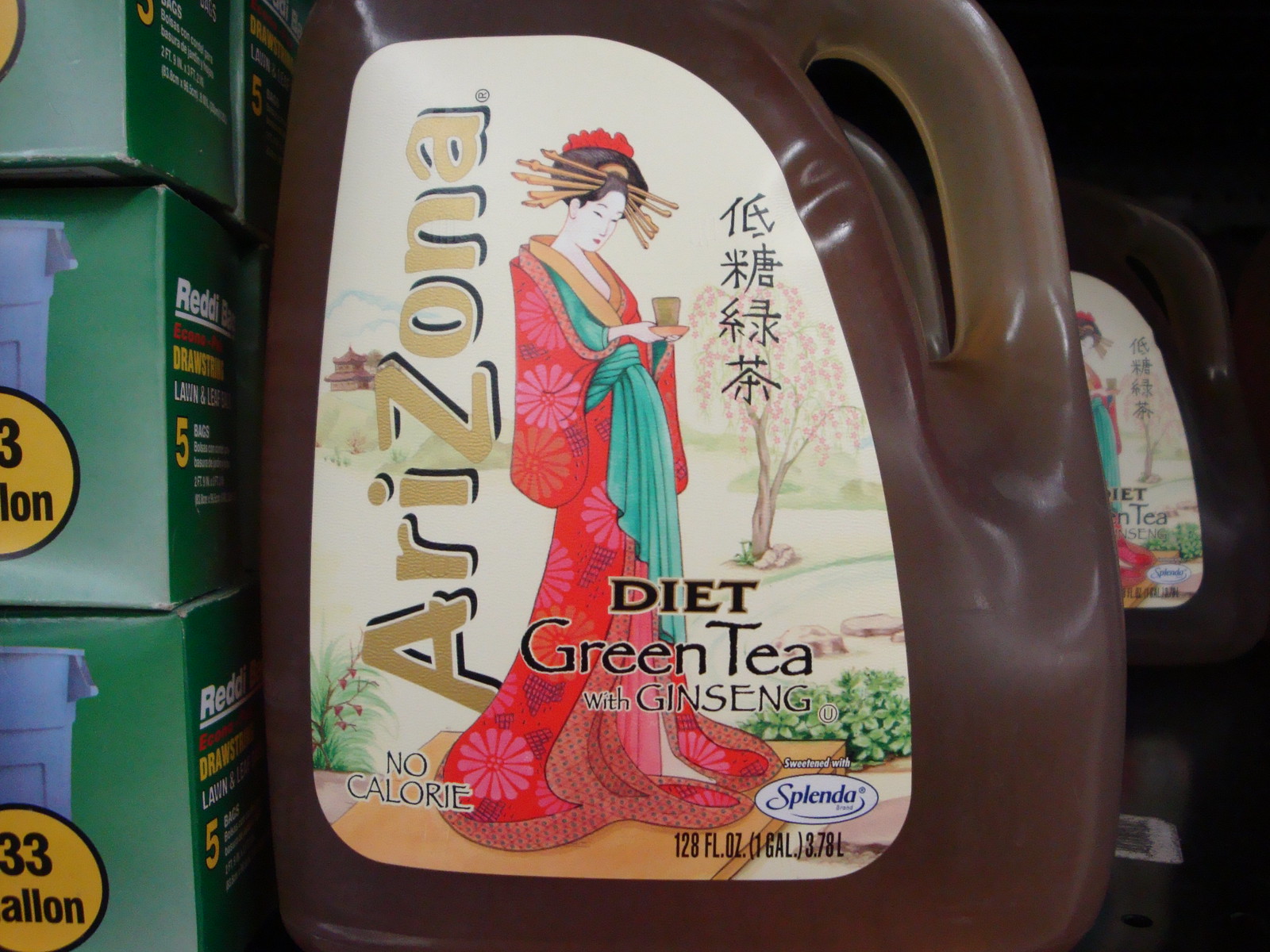This close-up photograph features a plastic jug of Arizona Diet Green Tea with Ginseng. The jug contains brown tea, visible through the transparent container. The label prominently displays "Arizona" vertically in gold letters against a white background. Also on the label is an illustration of a woman dressed in a red and turquoise robe, holding what appears to be a cup of tea. The bottom right-hand corner of the label contains the word "Splenda," indicating the type of sweetener used. Positioned behind this jug is another bottle of the same product, while adjacent to the jug, there are three stacks of green boxes, each containing drawstring 33-gallon trash bags.